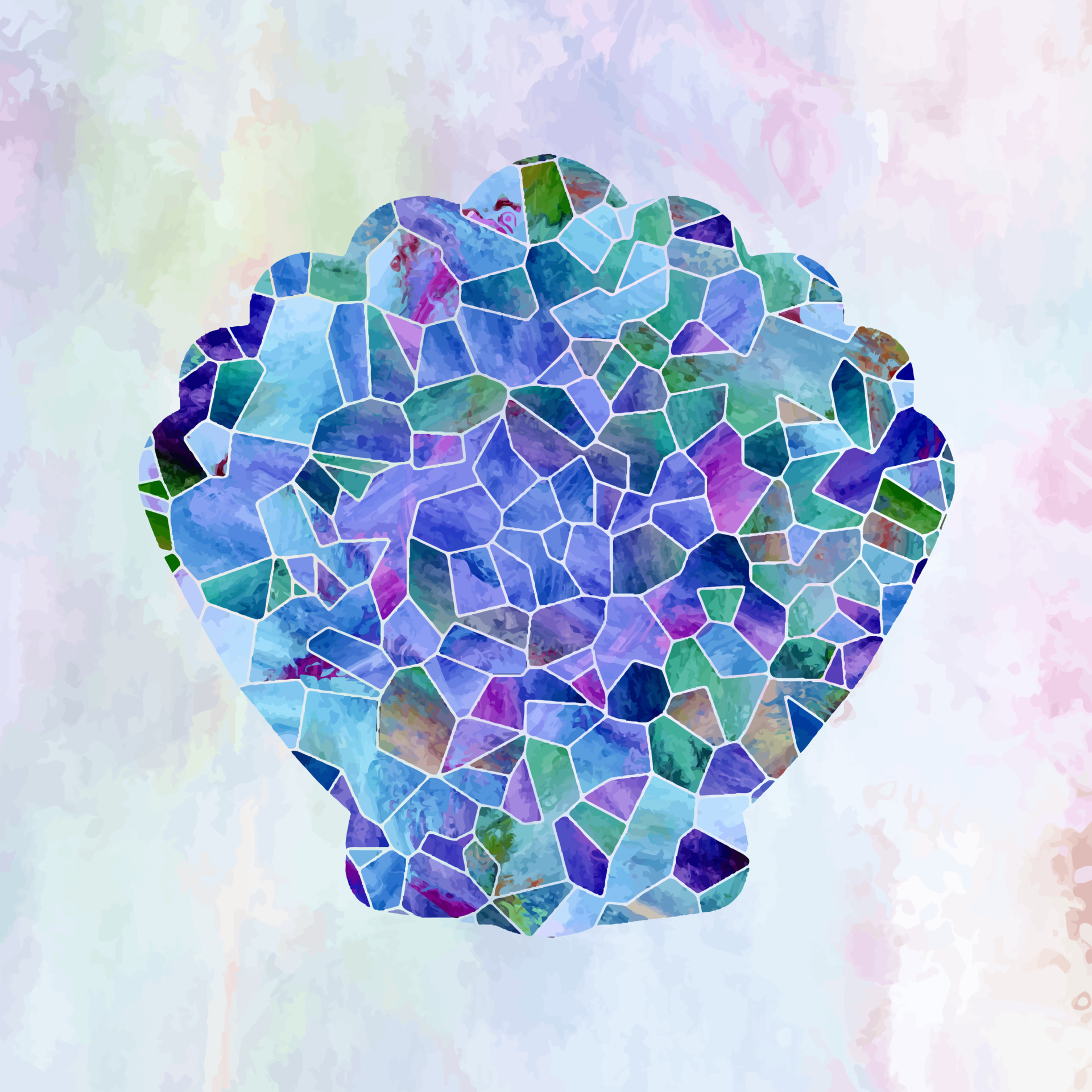This is a digital illustration of a seashell rendered in a stained glass or mosaic pattern, meticulously pieced together from various cool colors. The seashell, positioned at the direct center of the image, dominates the composition and is outlined in white, creating a segmented, puzzle-like appearance. The predominant colors within the seashell itself are marine hues, including blue, green, purple, and pink, with occasional touches of brown. Surrounding this central element, the background is a soft, pastel watercolor wash featuring shades of green, purple, pink, white, and some brown, applied in wispy, painted strokes. The overall look is flat and simple, offering a serene and harmonious blend of colors.